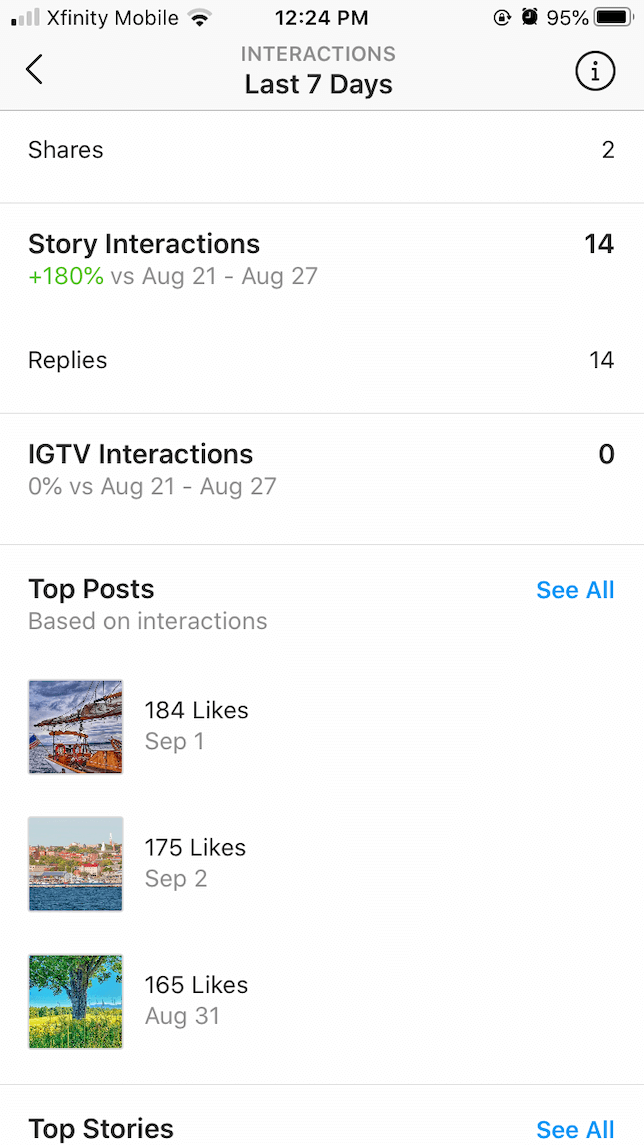This is a detailed screenshot showcasing an analysis of social media stories, possibly Instagram or a similar platform. At the top of the screen, the status bar shows signal strength through Xfinity Mobile, the time at 12:24 PM, an alarm icon, and a battery level at 95%. The primary heading reads "Interactions, Last 7 Days."

Under this heading, the metrics are broken down as follows:

- **Shares:** 2
- **Story Interactions:** 14 (highlighted in green with a +180% increase compared to August 21-27)
- **Replies:** 14 
- **IGTV Interactions:** 0 (indicating no change or activity, with 0% change versus August 21-27)

Below these metrics, a section labeled "Top Posts Based on Interactions" is displayed with a "See All" text link on the right. This section contains three thumbnail images with their respective details:

1. **A Sailboat:** 184 likes, posted on September 1st.
2. **A European Shoreline:** 175 likes, posted on September 2nd.
3. **A Tree in a Field:** 165 likes, posted on August 31st.

Further down, another section labeled "Top Stories" is present, again offering a "See All" option on the right. 

Overall, this screenshot provides a detailed breakdown of story interactions and top posts based on user engagement over the past week, helping to analyze social media activity, particularly the performance of shared stories and posts.